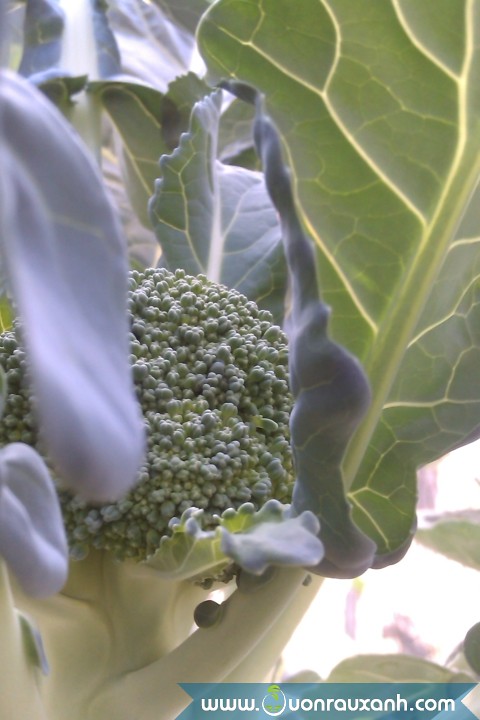The image showcases a highly zoomed-in view of a broccoli plant, characterized by its dark green, bushy head similar to the treetop of broccoli. The plant features thick green stems and is surrounded by large light green leaves, some tinged with purple. These leaves have clearly visible veins running through them. In the lower right-hand corner, there is an area of overexposed light, suggesting outdoor settings, possibly a garden, although the background details are minimal. The image includes a watermark directing to the website "wonrauxanh.com". Additionally, one of the stems displays a distinct bump resembling a caper.